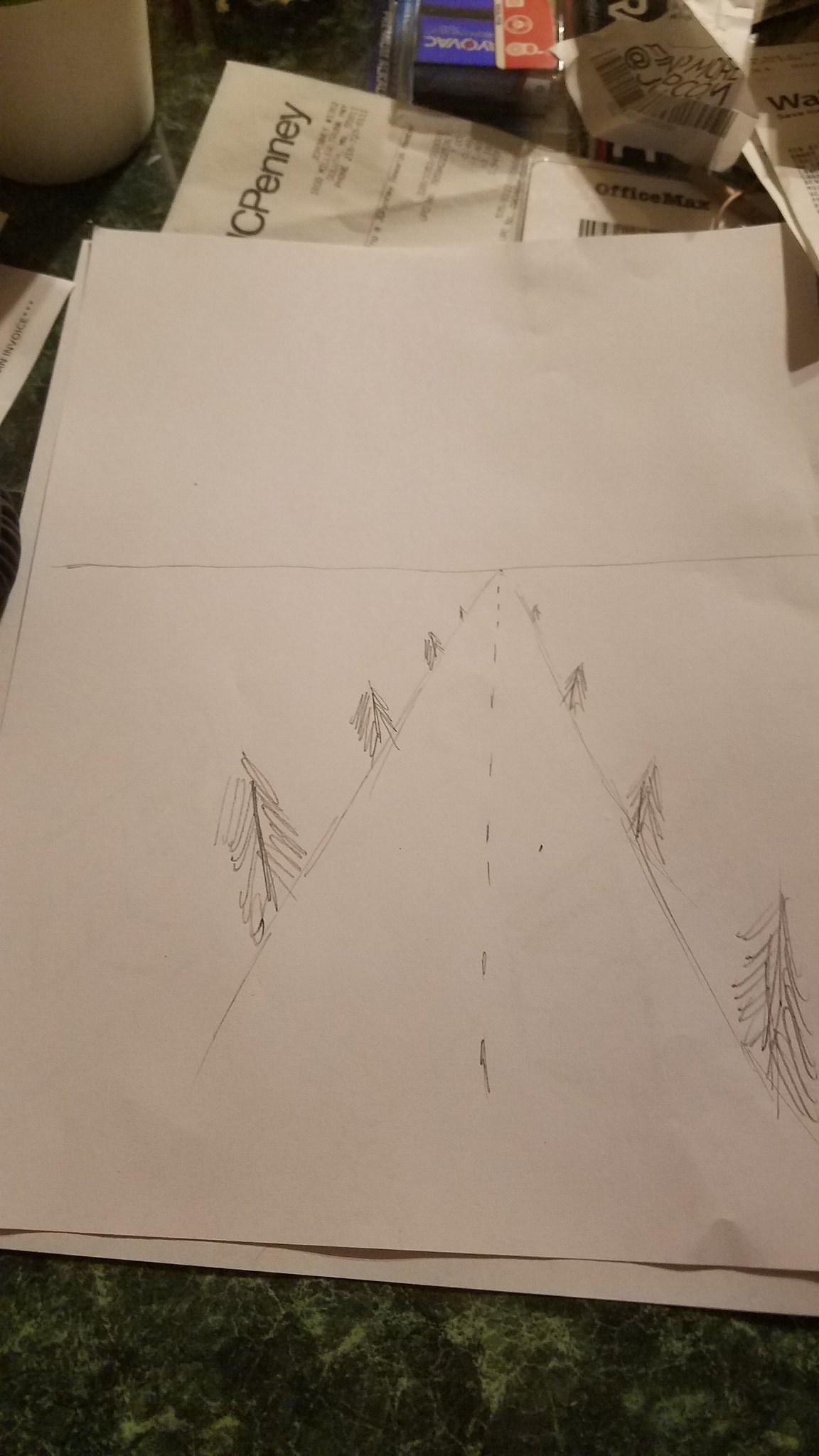The photograph depicts a cluttered green and white speckled marble countertop typical of an American household. Scattered across the surface are various items, including a white coffee cup, multiple receipts from stores like JCPenney and Walmart, packages of RailVac batteries, mail, a check or invoice, and a pencil sketch on a vertically oriented piece of white printer paper. The drawing, done by a child, features a two-way road with dashed lines running down the middle, converging at a vanishing point on the horizon along a horizontal line. Pine trees, characterized by vertical trunks and downward sloping branches, line both sides of the road.